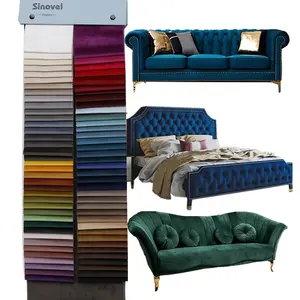This image is a composite advertisement featuring furniture pieces and a fabric swatch display. On the right, three pieces of furniture are showcased: a plush royal blue sofa with three throw pillows (two golden, one gray) at the top, a royal blue bed with a matching headboard and footboard in the middle, and a teal blue sofa at the bottom. To the left of these items, a swatch sample book, labeled "CINOVEL" in the upper left-hand corner, is displayed. This book contains around 100 fabric samples arranged in two columns, offering a wide array of colors from whites, neutrals, yellows, and browns to greens, purples, reds, blues, and grays. This setup appears to be part of an advertisement from a furniture outlet, indicating the available upholstery options for the featured furniture pieces.